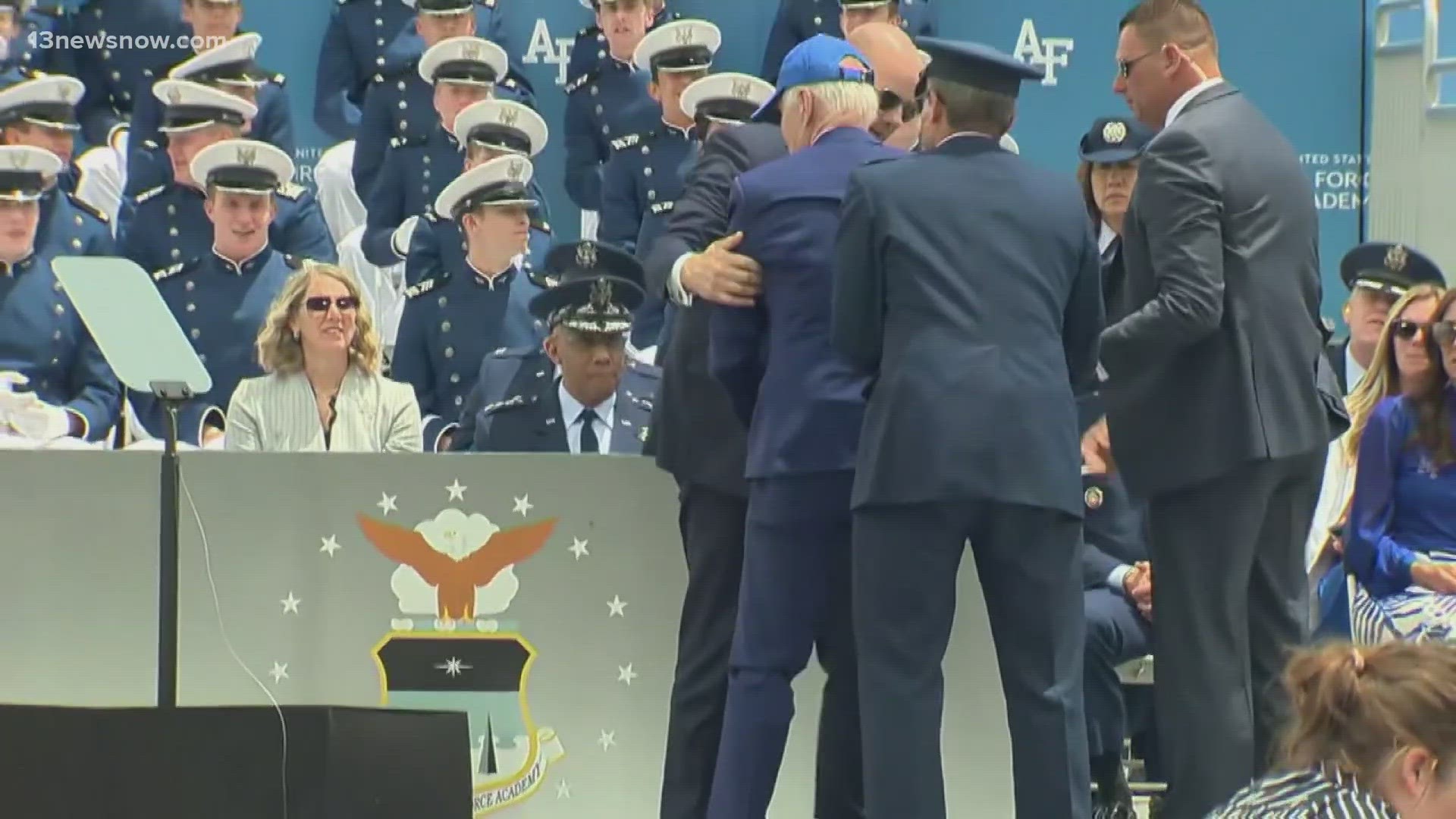In this photograph taken at an event likely held at the Air Force Academy, President Joe Biden is being escorted away from the stage by a group of Secret Service members after apparently tripping and falling. President Biden, viewed from behind, is distinguished by his blue suit and light blue baseball cap beneath which his gray hair is visible. A Secret Service member in a dark blue suit and hat stands directly behind him, while another member in a black suit with a visible white wire earpiece and short black hair, accompanies them. 

In the foreground, a bald man wearing sunglasses steadies Biden by placing his hands on the President’s arm. The backdrop includes a military audience seated in stadium-style seats, all dressed in blue uniforms with distinctive white caps featuring black brims and emblems. The scene is framed by a barrier separating the military personnel from the stage, and there's a notable appearance of a blonde woman in a white jacket and sunglasses among the attendees. Additionally, the stage features a podium and teleprompter screens, with the Air Force Academy symbol and related text visible, further indicating the specific context of the military event.